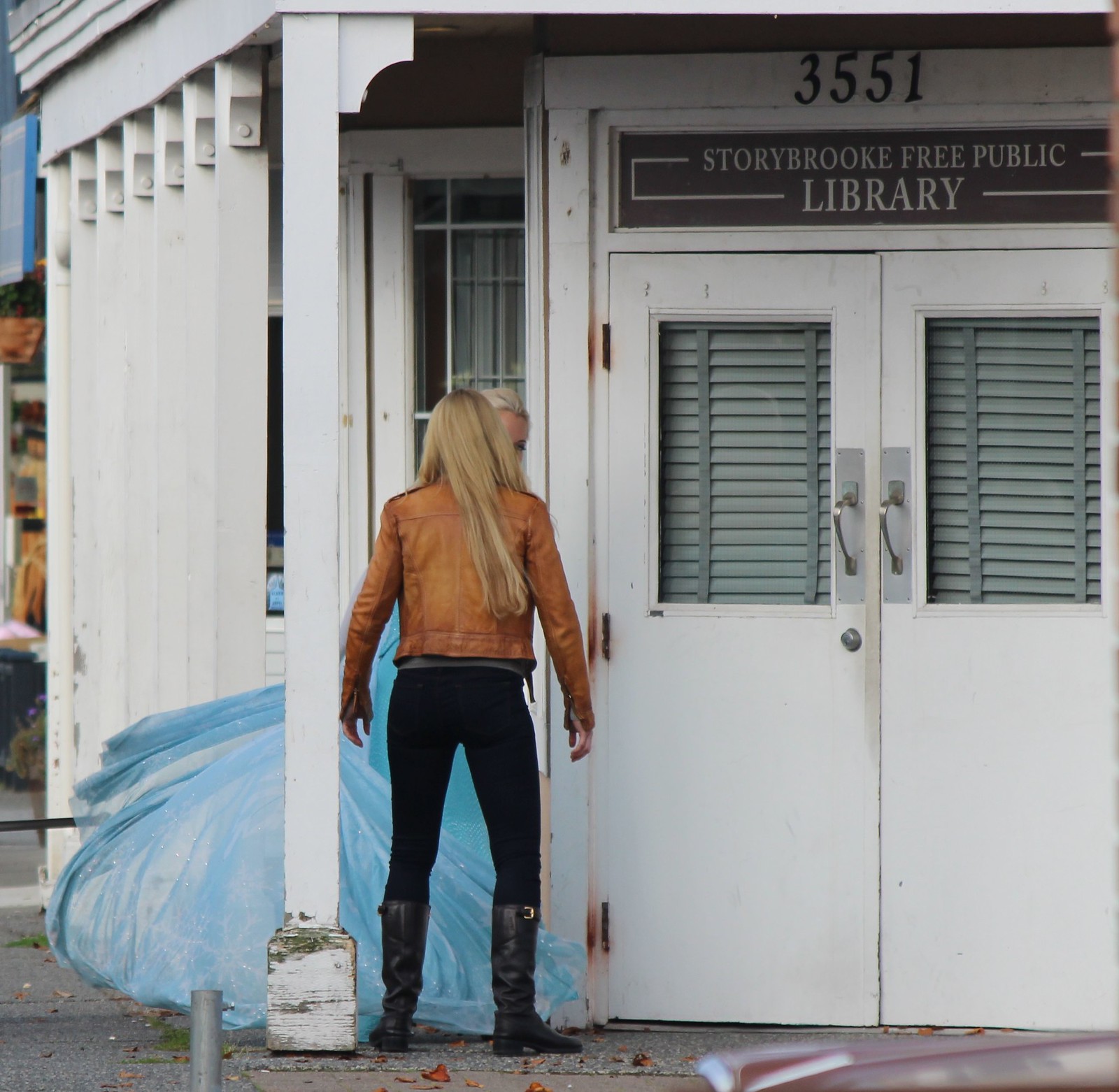In this image, two women stand outside a worn and rundown white building identified as the Storybrook Free Public Library, with the address 3551 prominently displayed. The building's façade shows signs of neglect, featuring rusted doors, tattered shades drawn over the windows, and weathered pillars supporting the roof. The women are positioned in front of the entryway, which includes windows on either side with closed shades. The woman with her back to the camera is dressed in an orange, suede-like jacket, black pants, and tall black boots with buckles. She has long blonde hair and stands with her arms slightly out to the sides, conveying an unhappy posture. Facing her is another blonde woman, partially obscured but noticeable for her elaborate blue dress with a flowing train, reminiscent of a Cinderella costume. The setting around them includes rundown sidewalks, emphasizing the neglected state of the area.